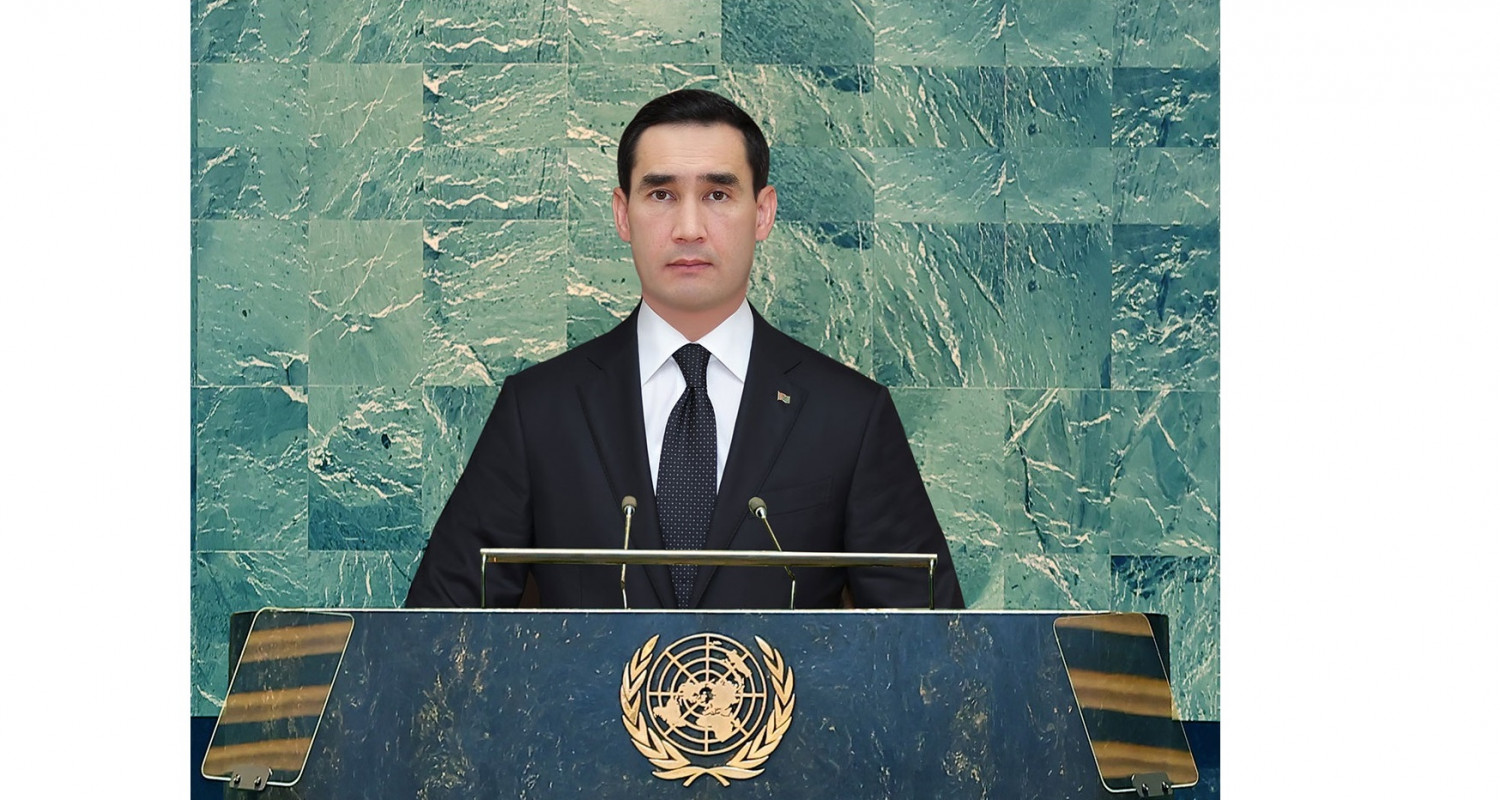This photograph showcases an Asian-looking man, likely the president of Turkmenistan, standing at a blue marble podium adorned with the golden emblem of the United Nations, featuring a globe encircled by two crisscrossed pieces of wheat. He is dressed in a black suit jacket with a white button-up shirt and a blue necktie adorned with white polka dots. A flag pin is affixed to the right side of his jacket. The man has short, dark hair and is clean-shaven, appearing to be in his 20s or 30s. 

In front of the podium are two small black microphones attached to a bar, flanked by what seem to be two clear glass screens. Behind him, the background consists of an intricate pattern of square, turquoise-green tiles with visible cracks, giving the impression of a stony texture. The man stands with a neutral expression, delivering a speech, though the specific occasion or event remains unclear.